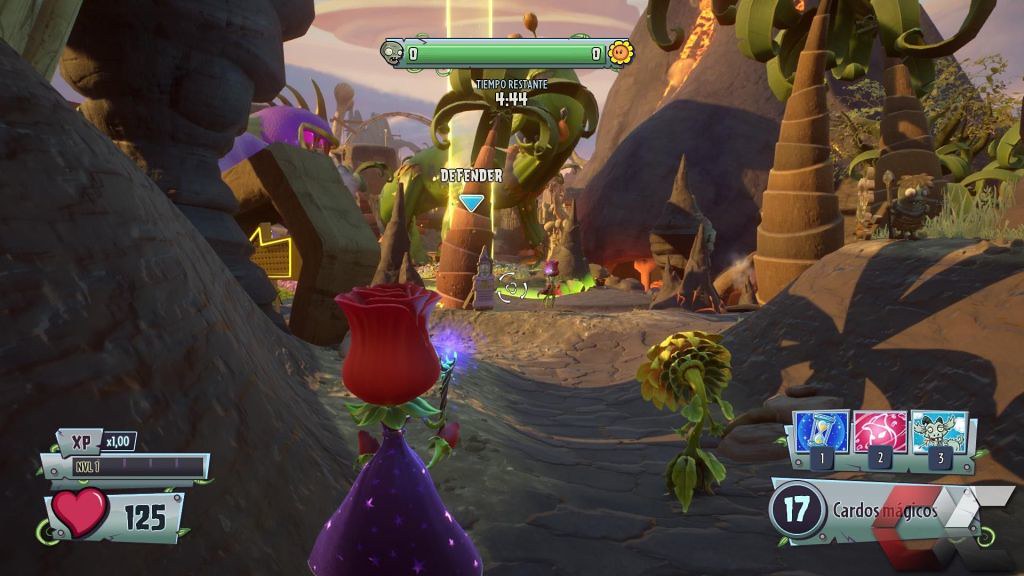In this vibrant and engaging snapshot from a video game, the ground texture resembles coarse, loose dirt. Embellished against a backdrop of towering, cartoonish palm trees and looming mountain peaks, a diverse array of animated characters populate the scene. Among these characters are whimsical humanoid flowers and figures resembling native people, the latter brandishing spears in a defensive stance. The bottom left corner of the screen features a rectangular interface element, prominently displaying a red heart icon alongside a score of 125. On the opposite side, in the bottom right corner, a circular interface piece marked with the number 17 adds to the visual storytelling and gameplay dynamics.